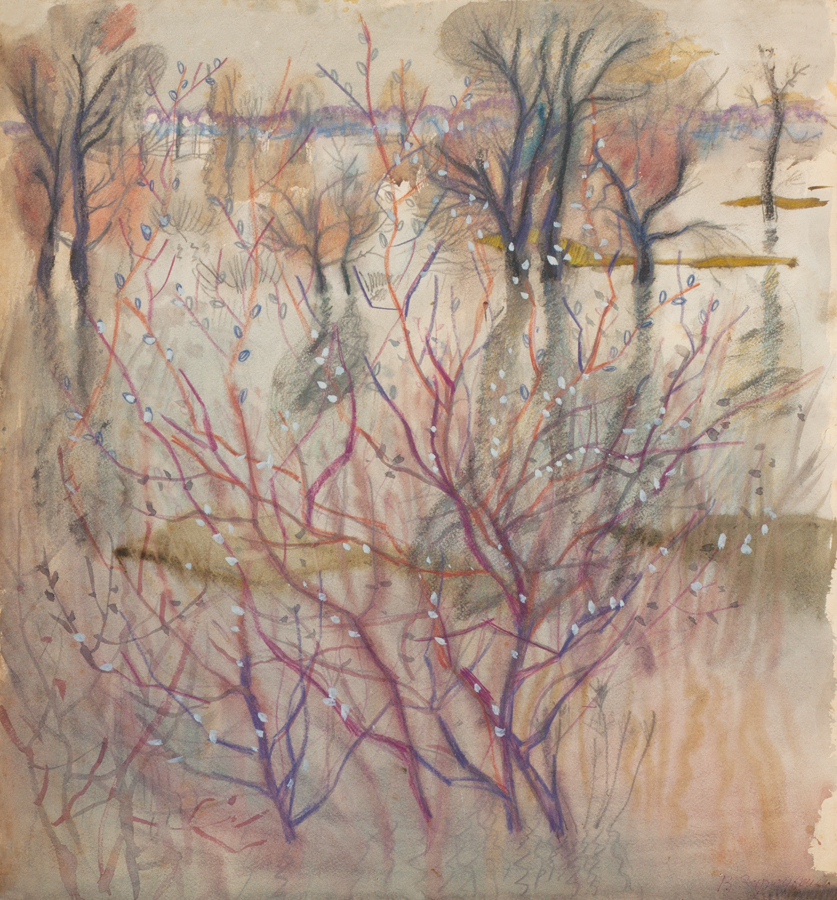This impressionistic mixed media painting vividly captures an autumn landscape scene, blending various artistic techniques. The background features a horizon line with soft, muted beige sky and small mountains tinged with a pink hue, overlooking blue waters. The larger areas seem to be rendered in delicate watercolors. Dotted across the landscape, trees exhibit a mix of techniques: their trunks and branches are likely drawn with dark chalk or oil pastels, creating a striking contrast with the watercolor backdrop. Fully grown trees appear in the background, surrounded by autumnal hues of red, orange, and yellow shrubbery at their base, evoking a shadowed, serene atmosphere.

In the foreground, barren trees with twisted branches stand starkly against the setting, with accents of reddish and bluish tones. These branches are adorned with small white dots, which could represent delicate leaves or flowers, adding an element of intrigue. At the base of these trees are lighter patches resembling soil or sand, enhancing the autumnal impression. The painting masterfully conveys the essence of a landscape transitioning through fall, with a dynamic interplay between water reflections and mixed media textures, creating an immersive, multi-dimensional effect.